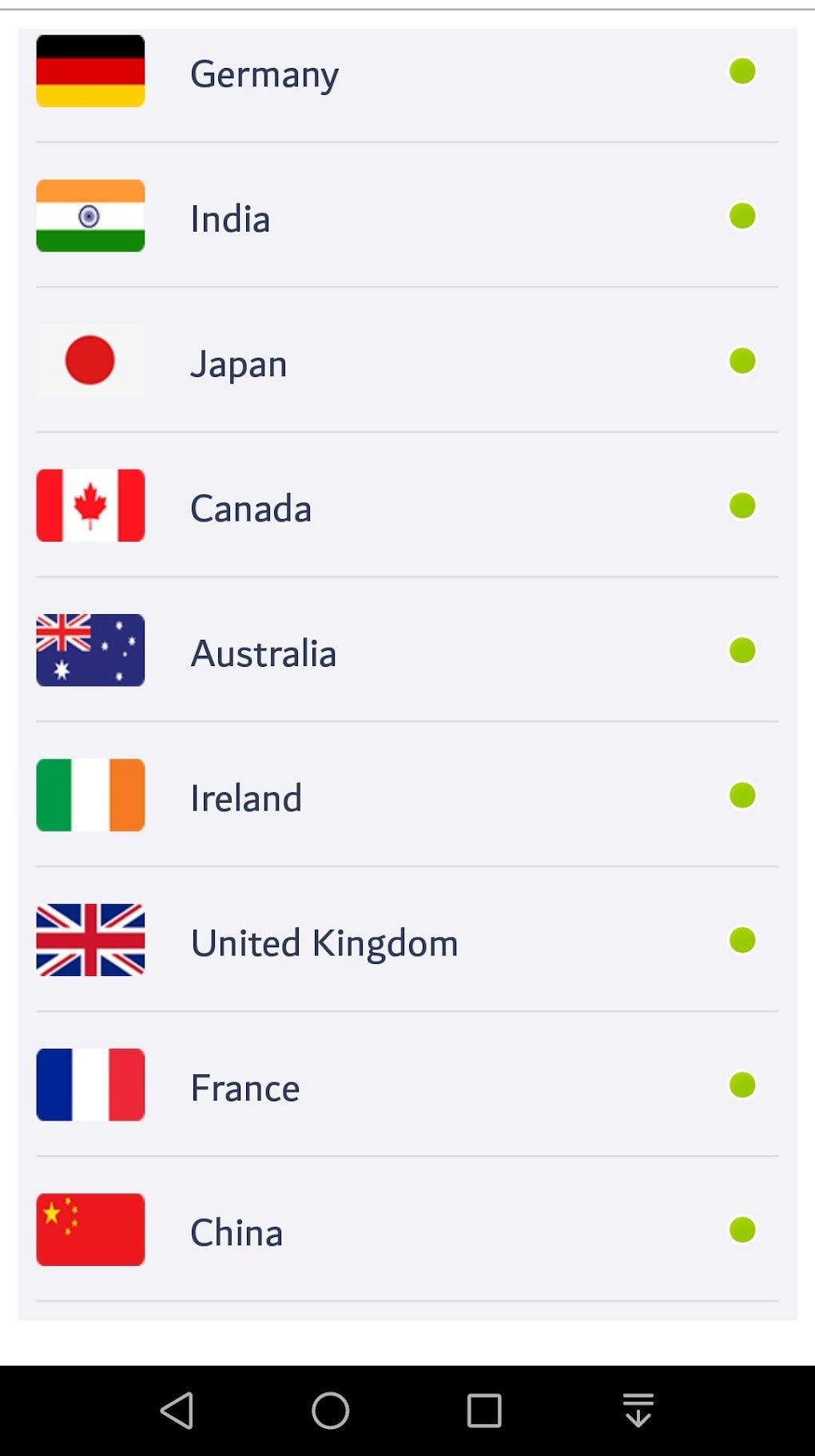This image is a cropped, full-color, computer-generated screenshot depicting a list of countries in a format that resembles a smartphone interface. The background is a soft beige, and the text, likely in Calibri font, is rendered in black for high readability. The list of countries is arranged vertically and includes Germany, India, Japan, Canada, Australia, Ireland, the United Kingdom, France, and China from top to bottom. Each country name is accompanied by its respective national flag positioned to the left. Beside each country and flag, there is a prominent green tick mark, suggesting that these countries might have been selected or marked off in some manner; however, it remains unclear if the tick turns black upon action or signifies pre-selection. At the very bottom of the image, navigation icons are visible, including a circular back button, commonly used to return to the home page, and a download button represented by two dashes and a downward arrow.